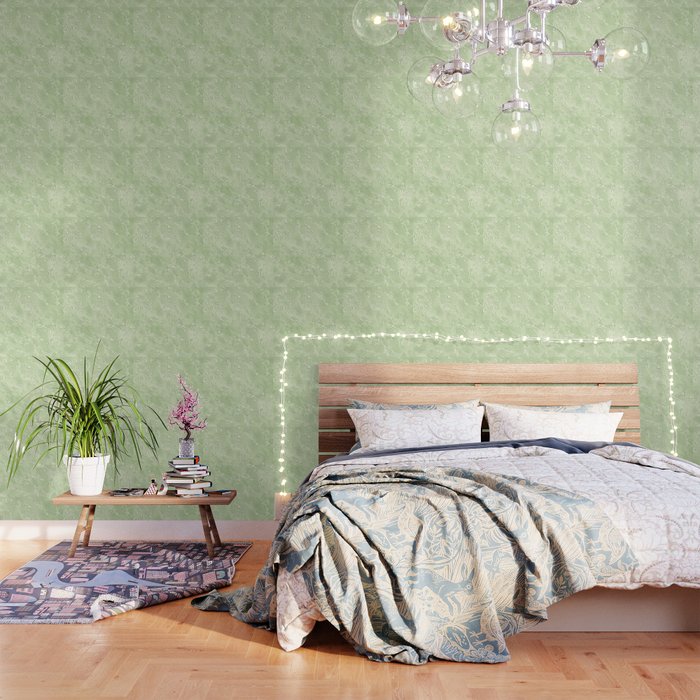This meticulously styled bedroom image, reminiscent of a high-end home decor magazine spread, captures an inviting, modern aesthetic. Dominating the scene, a low-profile bed adorned with a lavender comforter, matching shams, and four plump pillows sits in the bottom right corner. The bedspread is a light brownish color with a subtle pattern featuring animals such as rabbits and chickens, while the sheets offer a soft blue hue. Artistically tossed at the foot of the bed is a blue and white blanket, adding a touch of casual elegance.

The bed's headboard is made of horizontal wooden slats, resembling a charming fence design, and is accentuated by whimsical fairy lights outlining it, mounted a foot above the headboard on the green patterned wallpaper. This background exudes a calming vibe with its mint-green color and light, roundish patterns.

Suspended over the bed is a striking modern chandelier. Its silver base branches out into several crystal-clear globes, casting a soft, ambient light and drawing eyes to its futuristic design.

To the left of the bed stands a light brown bedside table at the same height as the bed. It holds a small stack of books topped with a vase containing a medium-sized plant with pink flowers, and next to it, another larger plant in a plain white pot. The table rests on a rectangular rug, which slightly disrupts the floor's harmony by being kicked up at one corner, hinting at a sense of lived-in comfort despite the room’s otherwise polished appearance.

The entire setup sits on a light brown wooden floor, pulling together various elements of color and texture into a cohesive, stylish, and inviting bedroom setting.